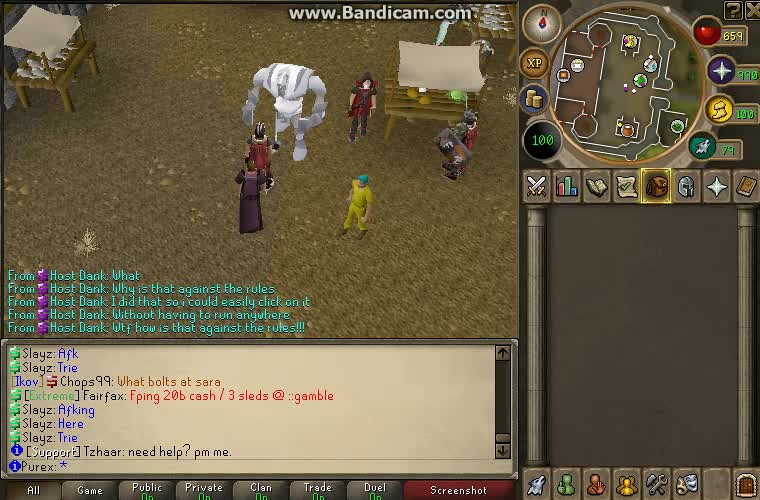This is a color screenshot of a classic RuneScape game, captured from a computer screen via Bandicam, as indicated by the text "www.bandicam.com" at the top center in bold white font. The interface mimics that of an online role-playing game, reminiscent of World of Warcraft in setup. 

In the top right corner, there is a circular mini-map, surrounded by various game stats including inventory icons for weapons, armor, notes, and journals. The main gameplay area extends to the left, featuring pixelated characters and a ground pattern of yellowish-brown dirt.

The bottom part of the interface houses the chat menu, where various players are communicating. Highlighted in this area, user Slays has written "AFK TRIE" in bright blue text, while other communications include user Chops99 asking "what bolts at Sarah?" and another user, Host Dank, discussing actions against the rules.

Below the chat menu are tabs for different chat categories like genre, public, private, clan, trade, duel, and screenshot. Various icons representing a wolf, a green person, a red person, a group of yellow people, and assorted weapons flank these tabs. Additionally, the top of the chat menu contains messages from another conversation involving a character expressing frustration over game rules.

Overall, the image depicts a richly detailed, nostalgic interface filled with typical MMORPG elements, making it instantly recognizable to fans of classic online role-playing games.